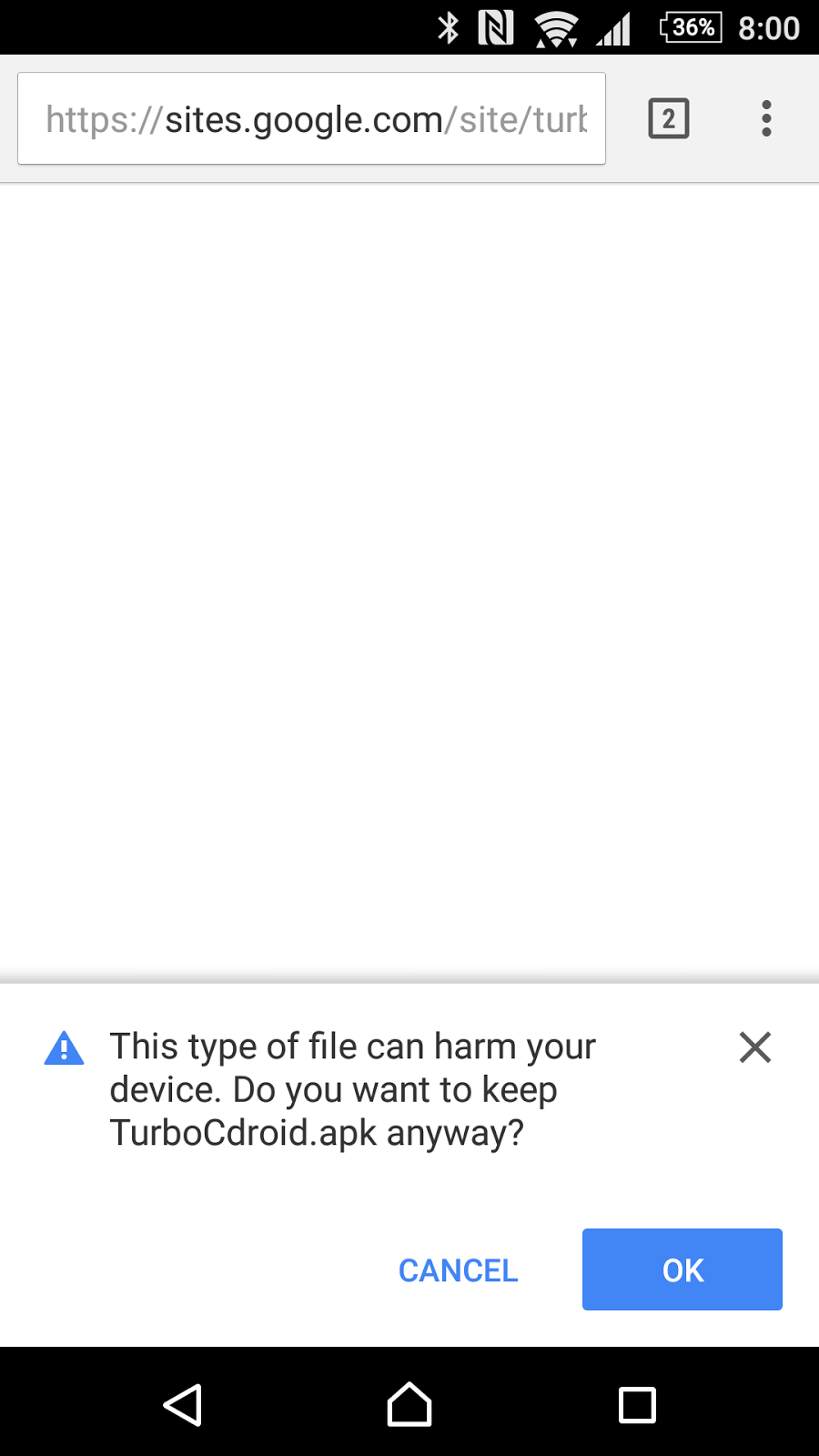This image, taken from a cell phone, captures a screen displaying a webpage URL: "https://sites.google.com/site-T-U-R-T". At the top of the screen, there is a tab indicator showing the number "2" within a box, and three vertically aligned dots are situated on the far right, indicating a menu or options button. The central portion of the screen is mostly blank and white, devoid of any content. Midway down, a horizontal gray line stretches across the entire width of the screen. Below this line, a security warning message appears: "This type of file can harm your device. Do you want to keep TurboCDroid.apk anyway?" There are two interactive options at the bottom of the message. The first is a capitalized blue text reading "CANCEL," and next to it, a blue button with "OK" in white letters. Adjacent to the warning message, there is a blue triangle containing a white exclamation point, signifying caution. At the very bottom of the screen, the standard navigation icons—a triangle, a house, and a square—are displayed within a black bar, each icon highlighted in white.